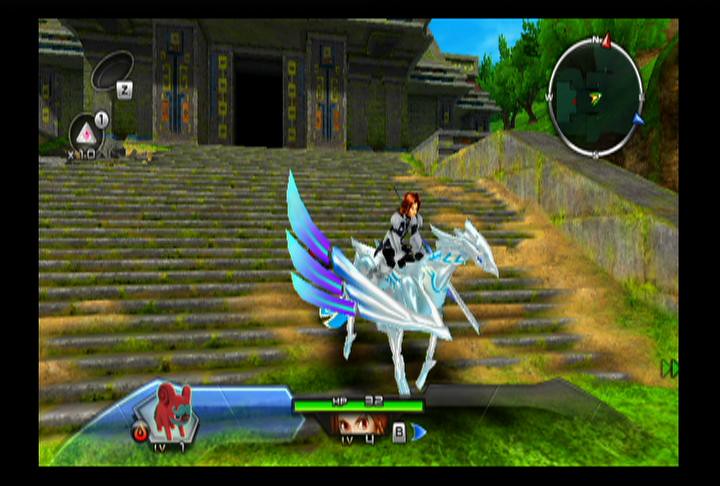The image captures an intense gameplay moment featuring a human character prominently positioned at the center. The character, with light brown hair, is donning a light gray top, and is depicted riding an enchanting creature. This creature is predominantly white, with a striking pair of wings adorned in gradients of light blue and purple. The creature's eyes are a mesmerizing blue, adding to its fantastical appearance. In the backdrop, a grand, endless staircase made of gray stone ascends into the distance, providing an epic and mystical atmosphere to the scene.